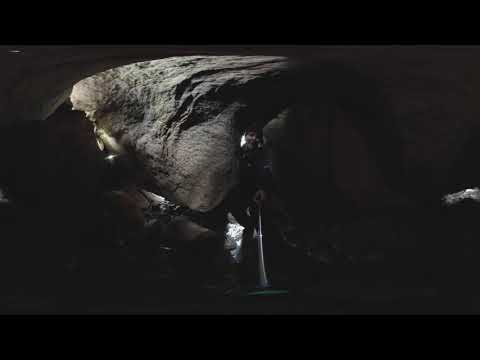The image captures a person, likely a woman, squeezing through a narrow, rocky crevice in what appears to be a cave or cavern. She is positioned in the center of the image, looking directly at the camera, which she seems to be holding with a selfie stick in her left hand. The surrounding rocks are large, weathered, and mostly gray to black in color, with a few lighter patches. Light filters into the scene from above and from the sides, illuminating parts of her body and the rock surface. She is wearing a black shirt, and a faint glimpse of the outside world is visible behind her through the gap. Her stance suggests she is making her way through a tight passageway, with one hand gripping what seems to be a flashlight or stick, adding to the sense of exploration in a dimly-lit, rugged environment.